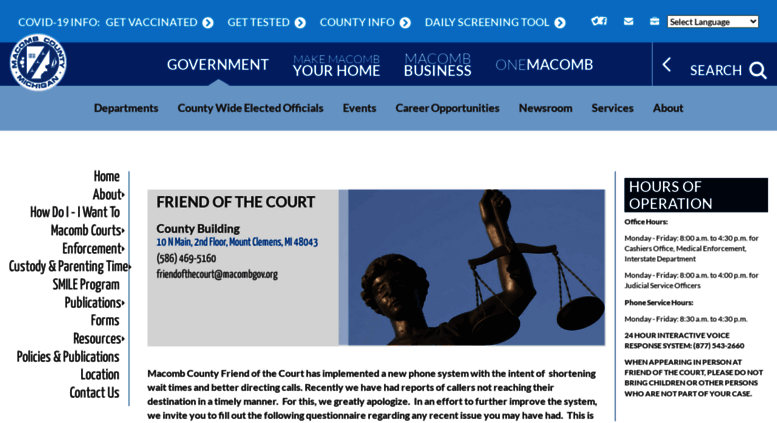The top part of this website features a light blue background with white accents. On the left-hand side, large capital letters announce "COVID-19 INFO" followed by a list of important actions: "GET VACCINATED, GET TESTED, COUNTY INFO, DAILY SCREENING TOOL." Below this, a white rectangle with a black outline houses the option to "SELECT LANGUAGE" in black text.

Continuing down, the background alternates between light blue and white. The words "GOVERNMENT," "MAKE MACOMB YOUR HOME," "MACOMB BUSINESS," and "ONE MACOMB" are displayed prominently. A vertical white line separates these sections from a search feature, which includes the word "SEARCH" in white alongside a white magnifying glass icon.

Further down, a darker blue background presents a series of department links in black text: "DEPARTMENTS, COUNTY-WIDE ELECTED OFFICIALS, EVENTS, CAREER OPPORTUNITIES, NEWSROOM, SERVICES, ABOUT."

The lower section features a white background. A vertical bluish line on the left side separates the main content, listing links in black text: "HOME, ABOUT, HOW DO I, I WENT TO MACOMB COURTS, ENFORCEMENT, CUSTODY AND PARENTING TIME, SMILE PROGRAM, PUBLICATION, FORMS, RESOURCES, POLICY AND PUBLICATIONS, LOCATION, CONTACT US."

Adjacent to these links is an icon of the "Justice is Blind" symbol, depicting Lady Justice holding scales. Below this icon, in black text, the website mentions the "FRIEND OF COURT, COUNTY BUILDING" with further details in blue: "10 North Main, Second Floor, Mount Clemens, MI 48043." Additionally, a phone number is listed in black: "586-469-5160" along with an email address: "friendsofcourt@macombb.org."